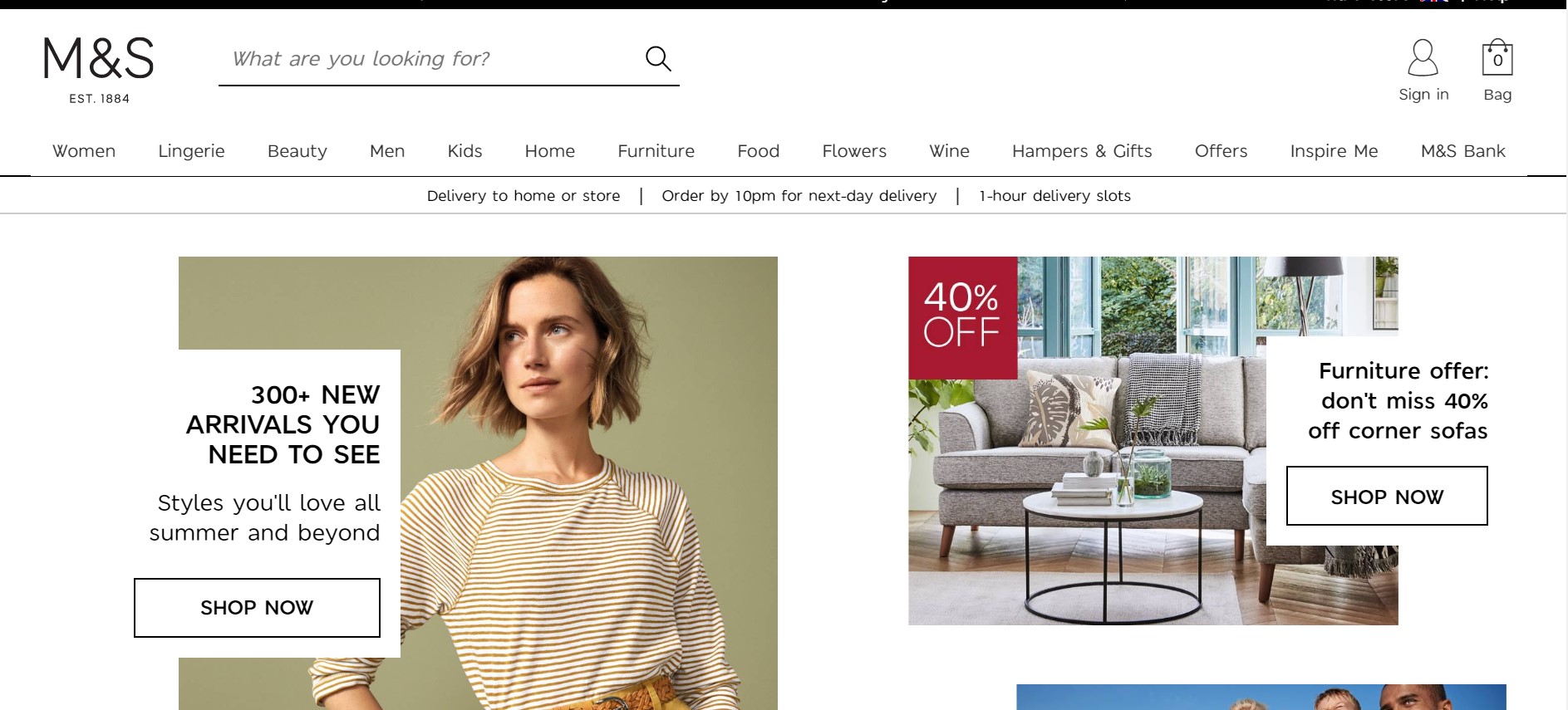This screenshot represents the upper section of the homepage for M&S, a renowned retailer established in 1884. At the top, it features the M&S logo alongside a search bar prompting, "What are you looking for?" To the right, there are icons for sign-in and a shopping bag. The primary navigation includes categories such as Women, Lingerie, Beauty, Men, Kids, Home, Furniture, Food, Flowers, Wine, Hampers & Gifts, Offers, Inspire Me, and M&S Bank.

Beneath the navigation bar, a service note reads: "Delivery to Home or Store, Order by 10pm for next day delivery, 1-hour delivery slots." Below this, promotional banners appear. On the left, a stylish woman stands against a beige background, wearing a brown-striped top and glancing off-camera. Adjacent to her, a message highlights "300+ new arrivals you need to see, styles you'll love in the summer and beyond," accompanied by a "Shop Now" button.

To the right, an image showcases a living room setting with a grey couch adorned with cushions and a glass-topped coffee table, advertising a remarkable "40% off corner sofas" deal, which also includes a "Shop Now" button.